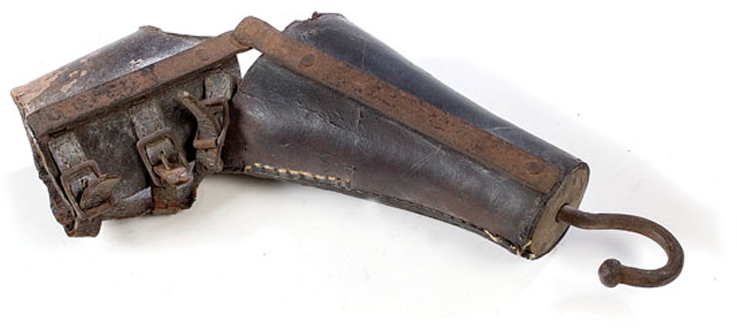The image depicts an old, rustic gun holster made of brown leather, prominently featuring a rusted metal hood at its head on the right side. The holster is aged and weathered, adorned with two rusted metal panels joining its upper and lower parts. Toward the bottom left of the holster, there are three horizontal stripes and two additional separate stripes. The overall colors in the picture range from rusty brown to pale yellowish-white and dark brownish-black. The holster is positioned slightly bent from the middle left towards the middle right against an empty, white background, evoking the sense of a worn, vintage piece of equipment.